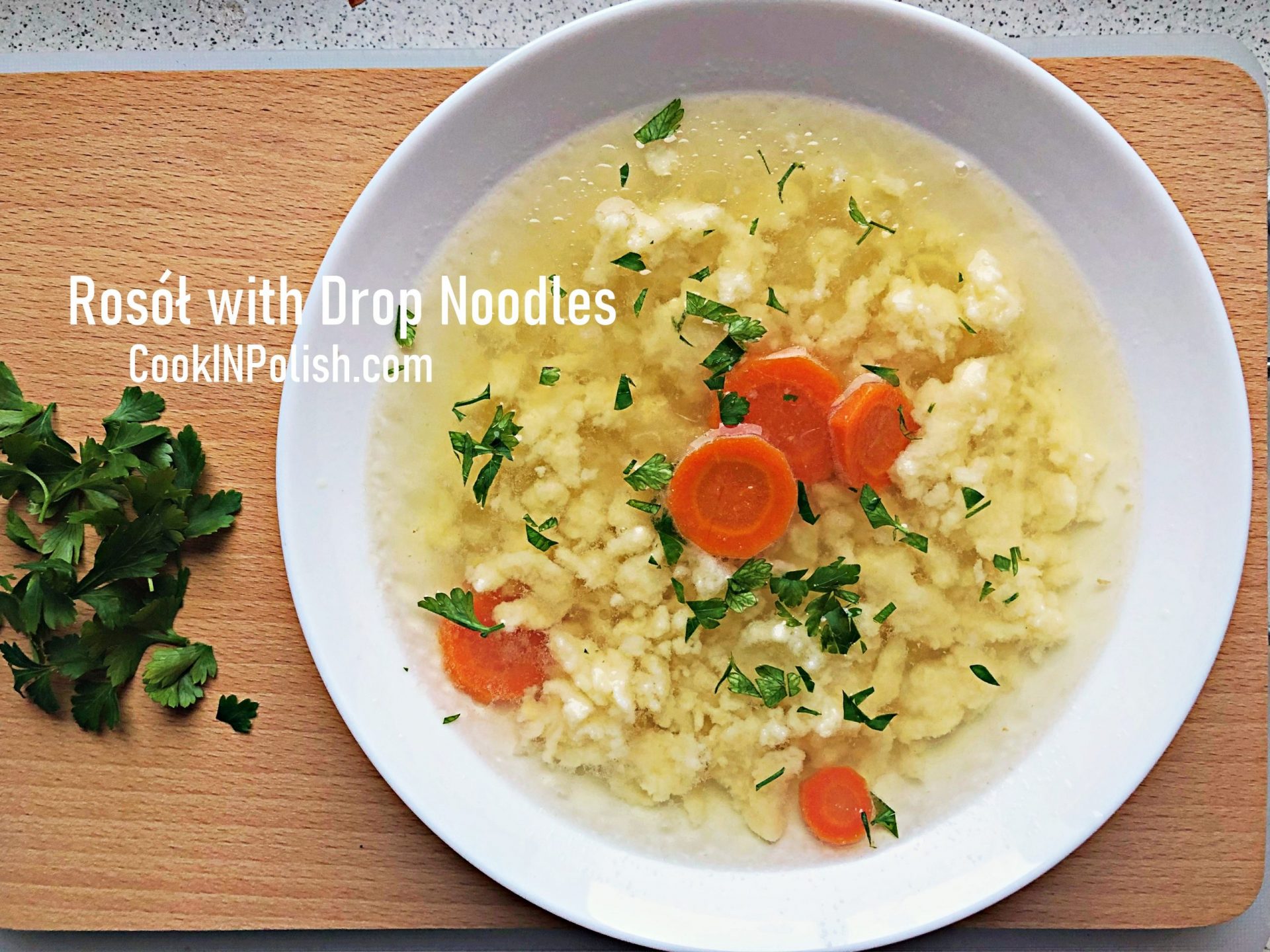The image displays a bird's-eye view of a bowl of Polish drop noodle soup, identified by text reading "ROSOŁT" and "cookinpolish.com." The soup, served in a deep white bowl, features small, white, textured noodles submerged in a light yellow, clear liquid. Accompanying the noodles are five round slices of carrots and a sprinkling of fresh green herbs, likely basil, adding a touch of color to the dish. On the left side of the image, finely chopped green herbs are placed beside the bowl. The scene is set against a wooden table, enhancing the homey and rustic presentation of this traditional Polish dish.